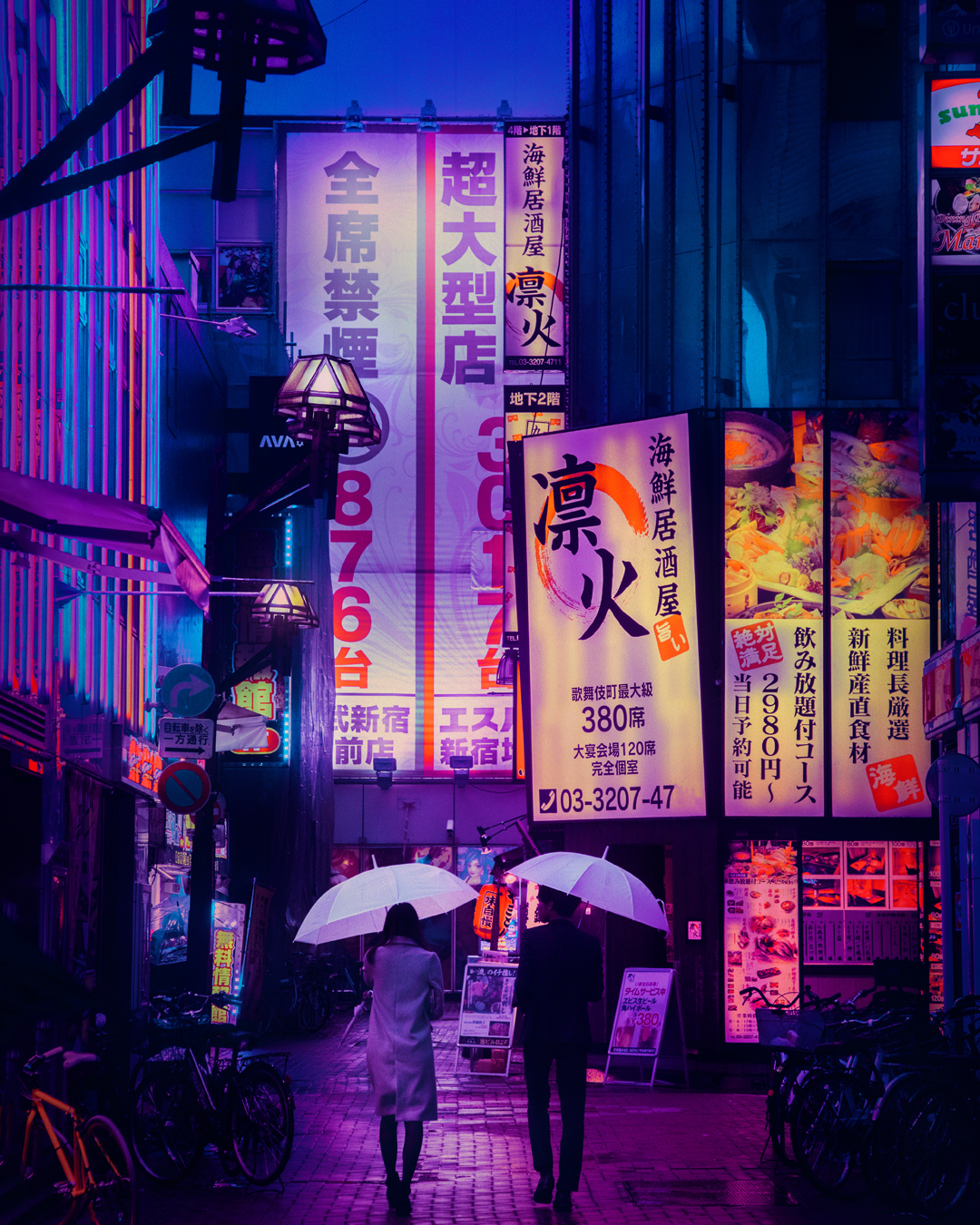The nighttime photograph captures a vibrant urban scene in an Asian city, possibly Japan. The image is bathed in a striking color scheme of purples and blues, illuminated by neon-bright signs and billboards that feature a mix of advertisements for food and various establishments written in Asian characters, potentially Chinese or Japanese. The backdrop includes tall buildings with white-lit, red, and purple inscribed billboards, contributing to the radiant atmosphere. 

On the cobblestone sidewalks, which glisten as if wet from recent rain, numerous bicycles are parked both on the left and right sides of the walkway. The focal point of the image is a couple seen from behind, walking and sharing a white umbrella. The woman is dressed in a gray coat that reaches her knees, accompanied by black leggings and black shoes, while the man is attired in a sleek black suit. The brightly lit restaurant window to their right displays enticing images of Chinese cuisine, further enriching the scene with cultural context and culinary allure.